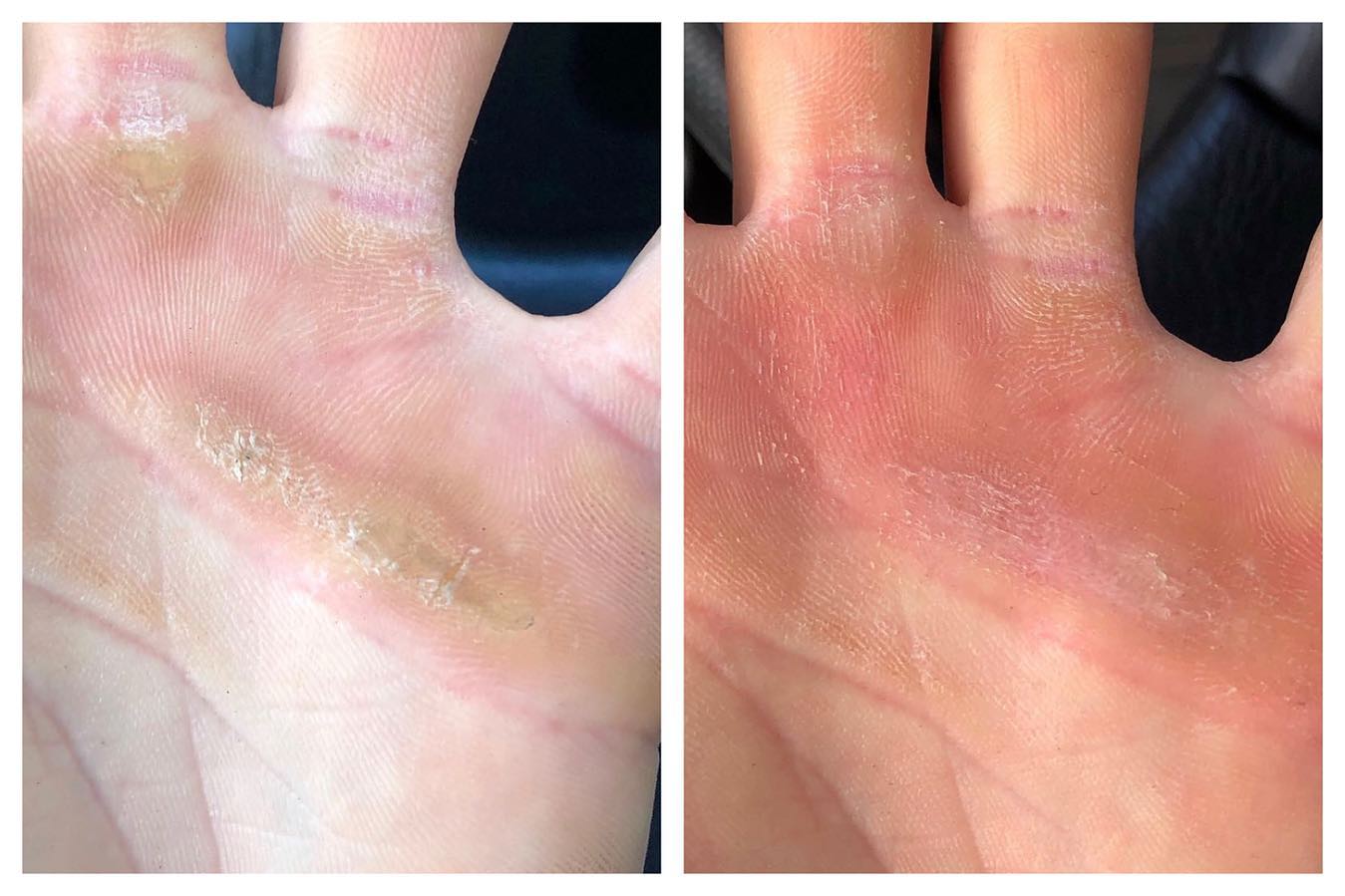The image set comprises a pair of detailed close-up photographs depicting a Caucasian adult male’s left palm before and after a dermatological treatment for skin calluses. The first photo shows the hand with severe calluses spanning the ball of the palm and extending to the base of the middle, ring, and pinky fingers. The skin appears dried and hardened, highlighting a pronounced rough texture. The subsequent image portrays the same hand post-treatment, exhibiting a noticeable reduction in the calluses, featuring a smoother surface with residual redness, suggesting recent skin recovery. Both photographs are set against a stark black background, punctuating the bends of the knuckles and the overall changes in skin condition.